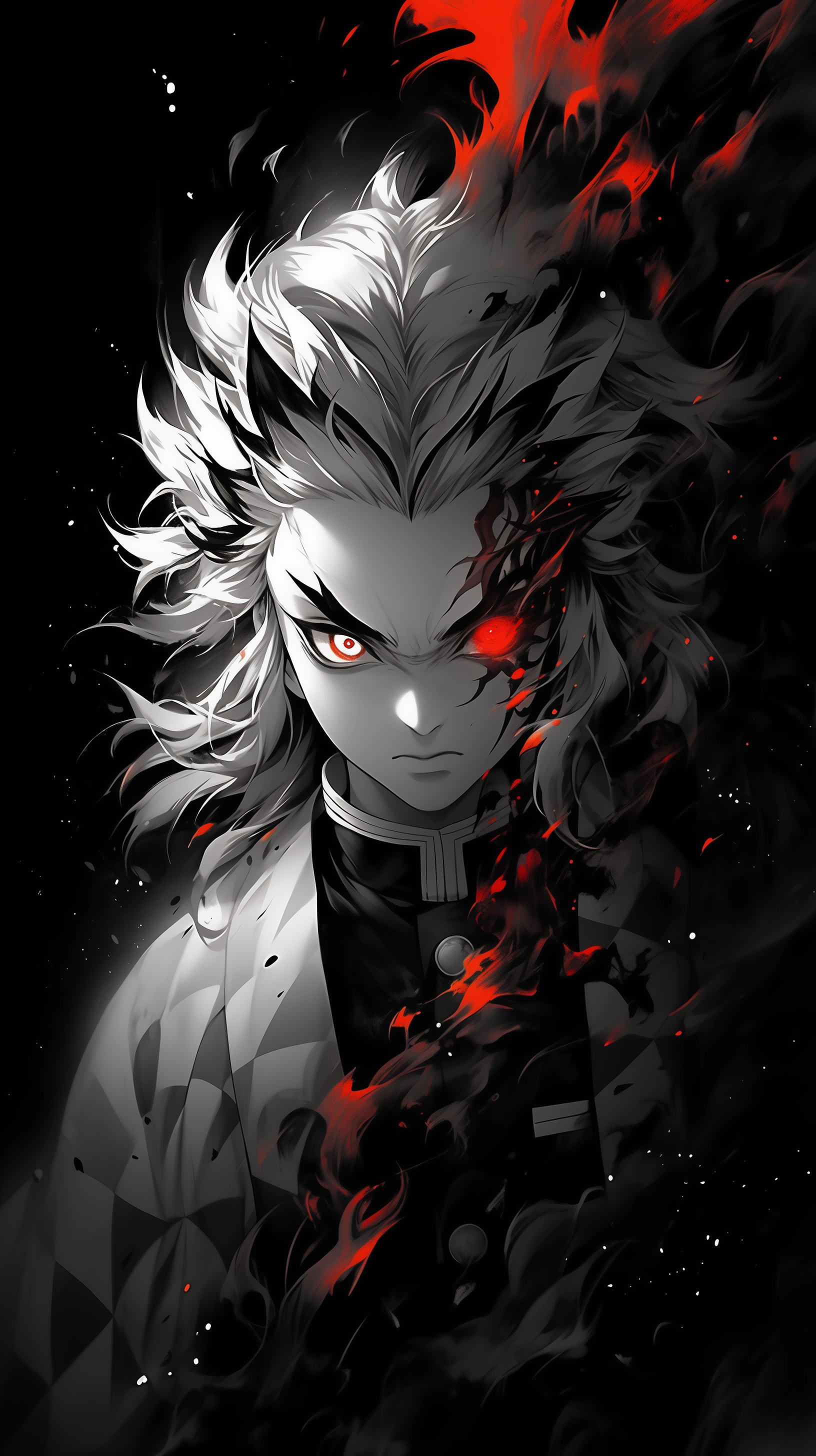The image depicts a striking anime character set against a solid black background sprinkled with white speckles. The character, shown from the torso up, has an intense and edgy appearance. This predominantly monochrome figure features wild, long hair reminiscent of a lion’s mane, predominantly white with black-tipped edges. His hair appears to be blowing as if caught in a wind, adding to the dynamic feel of the illustration.

The character's face is marked by a scowl, with thick black eyebrows enhancing his intense and pissed-off expression. His right eye is entirely red, with black and red vein-like marks extending from the bottom left to the top right, lending a possessed, demonic aura. The left eye, in contrast, is white with a red outline and a red pupil, glowing ominously. Red and black markings also trail across the right side of his body, further emphasizing the sinister effect.

Illuminated from the left side, the character's pale skin reflects the light, enhancing the stark contrast of his features. He wears a black and white collar and a multicolored jacket that resembles a military uniform over a traditional Japanese high school uniform. The overall composition, combined with the character’s elaborate hairstyle, fiery eye, and intense frown, creates a captivating and formidable image.